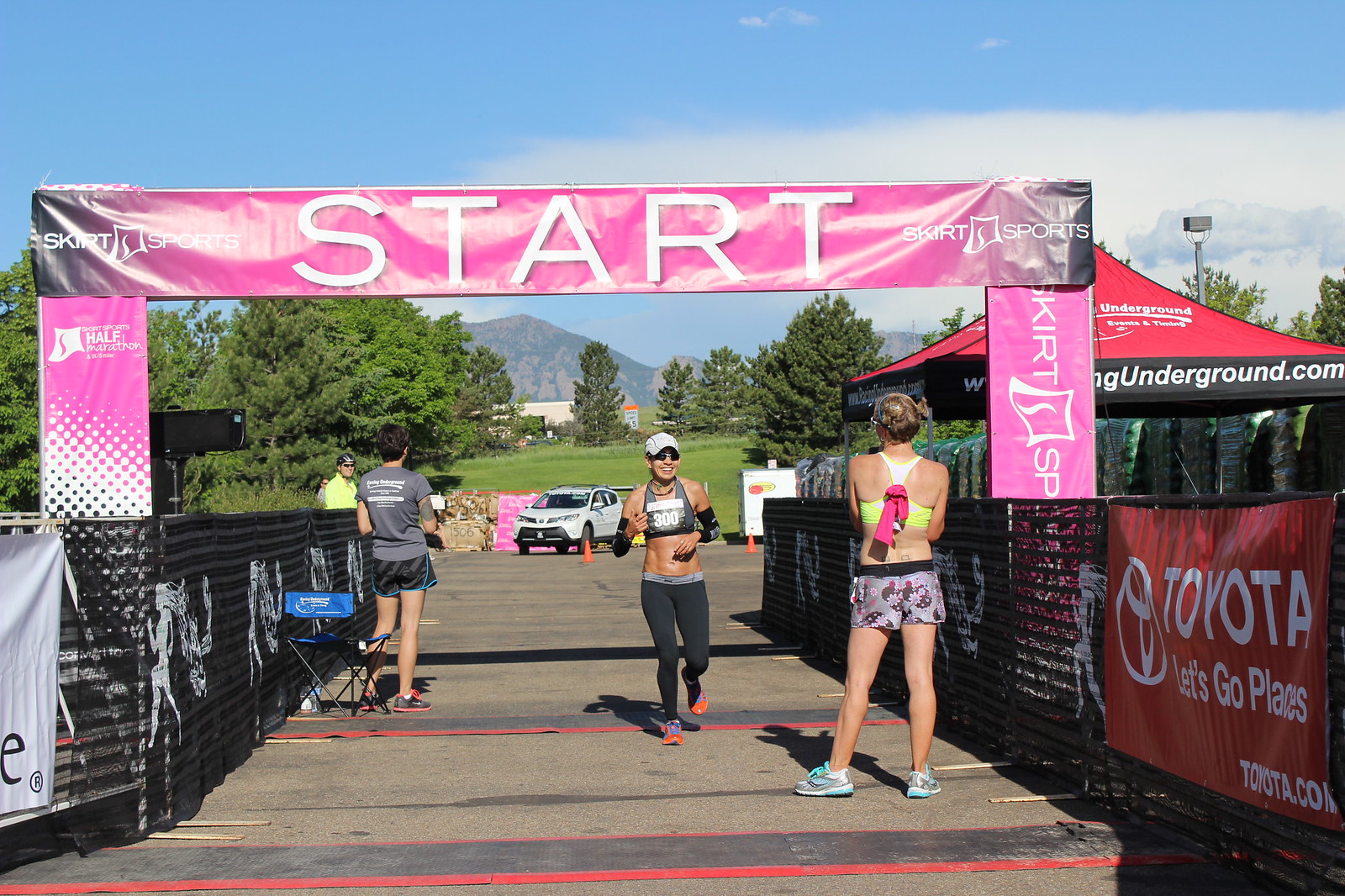The image depicts the bustling starting line of a Skirt Sports half marathon, predominantly featuring female runners. A prominent pink ribbon arching across the top, boldly labeled "START," spans the starting gate supported by sturdy pillars marking the occasion. The left pillar announces "half marathon," while the right reiterates "Skirt Sports," and both sides feature a red banner proclaiming the sponsorship of "Toyota - Let's Go Places." 

The scene unfolds on a blacktop parking lot, enclosed by black webbed fencing, which ensures a clear pathway for the runners. Center stage, a woman steps energetically under the start sign. She is dressed in black leggings, a matching sports bra with the race number "300," a gray baseball cap, and sunglasses. Adjacent to her, on the right, another woman clothed in neon green sports bra and short gray running shorts, with blonde hair, looks back, possibly sharing an encouraging glance.

In the background, adding to the lively scene, a few other participants mill around. One woman, dressed in a halterback tank top, shorts, and running shoes, stands prominently, while another, adorned in leggings, sports bra, arm braces, and orange shoes, greets someone with a smile. The image is framed by the dynamic interaction and the high-energy anticipation typical of race day beginnings.